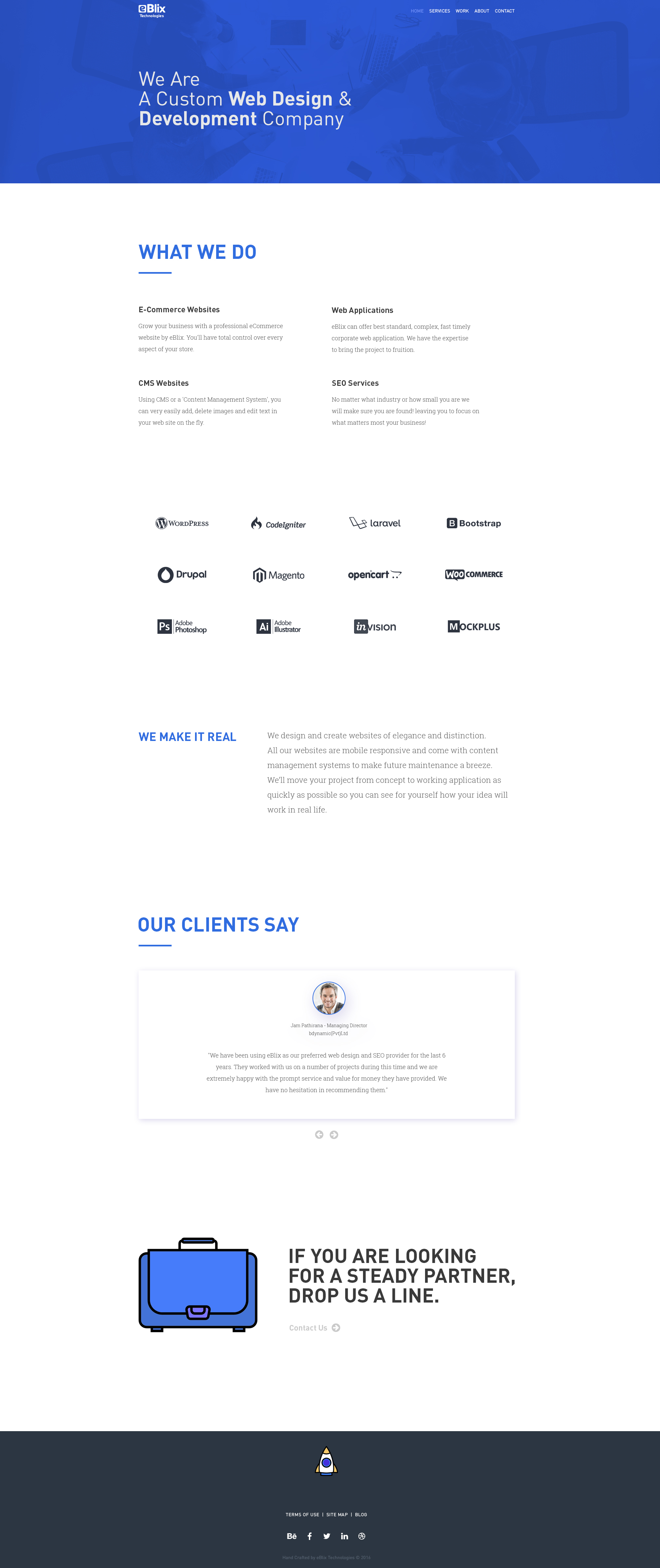At the top of the image, there is a dark blue header featuring the text "A Custom Web Design and Development Company" in bold white letters. Directly below, in bold blue capital letters, it states "WHAT WE DO," underlined for emphasis. Following this header, the text "E-commerce Website" appears in black. Below, in gray text, it reads, "Grow your business with a professional e-commerce website. Something you'll love and have total control over every aspect of." The smaller text beneath this is mostly unreadable despite zooming in. The subsequent sections list services including "Web Applications," "CMS Website," and "SEO Services," with each term presented in black text.

Near the bottom, there is a collection of logos representing various brands and technologies, including WordPress, Drupal, Adobe Photoshop, Magento, InVision, Mockplus, Bootstrap, WooCommerce, and OpenCart.